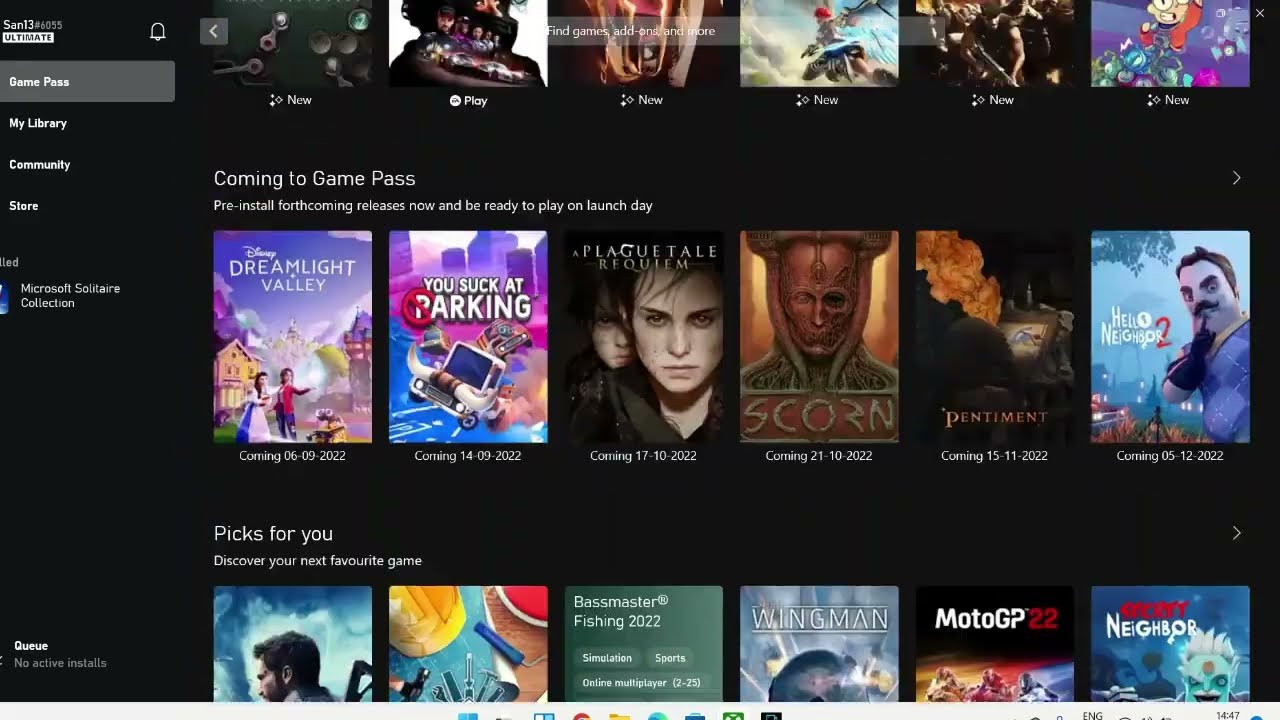This image features a close-up view of a digital interface on a tablet or computer screen, possibly showcasing a gaming service platform. In the upper left-hand corner, there is a label that reads "San 13 number 6055, Ultimate," likely referring to a user identifier or subscription tier. Below this, a navigation bar lists options such as "Game Pass," "My Library," "Community," and "Store." The primary focus is on the "Microsoft Solitaire Collection" title, positioned prominently and suggesting it is a featured game.

The interface displays an assortment of game images, vividly colored against a black background with white text detailing game titles. The game titles visible include "The Dreamlight Valley," "You Suck at Parking," "The Plague Tale Requiem," "Scorn," "Pentament," and "Hello Neighbor 2." There are additional thumbnails at the bottom whose titles are partially obscured. All in all, 18 game images are displayed on the screen, making for a vibrant, visually stimulating array that effectively highlights the variety of games available through this gaming service.